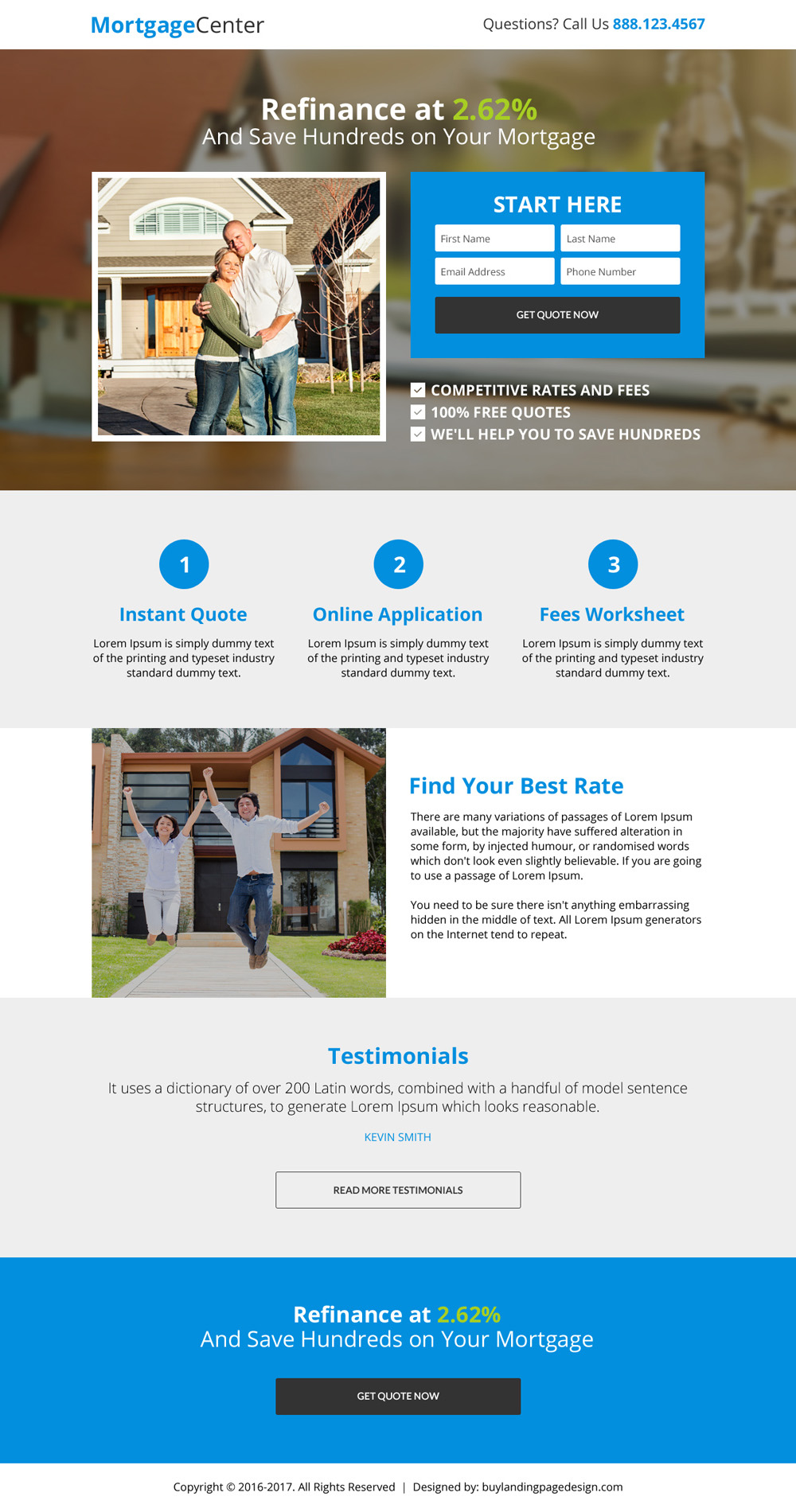The image depicts a homepage of a mortgage website. In the top left corner, "Mortgage Center" is prominently displayed with "Mortgage" highlighted in blue. In the top right corner, there is a contact number, "Questions? Call us 888-123-4567." 

Below this header, there is a main section featuring a blurred background image overlaid with a clear picture of a smiling man and woman embracing in front of a house. The house is characterized by light brown walls and a bright wooden door. Above this image, text reads: "Refinance at 2.62% and save hundreds on your mortgage."

Adjacent to the photo on the right, a small box labeled "Start Here" contains a simple form with four fields: "First Name" (top left), "Last Name" (top right), "Email Address" (bottom left), and "Phone Number" (bottom right). Beneath these fields, a button labeled "Get Quote Now" invites user interaction.

Further down, three small informational squares are lined up horizontally. The first square reads "Competitive Rates and Fees," the second says "100% Free Quotes," and the third claims "We'll Help You to Save Hundreds." Below these squares, a three-step process is outlined with the numbers 1, 2, and 3, detailing "Instant Quote," "Online Application," and "Fees Worksheet" respectively.